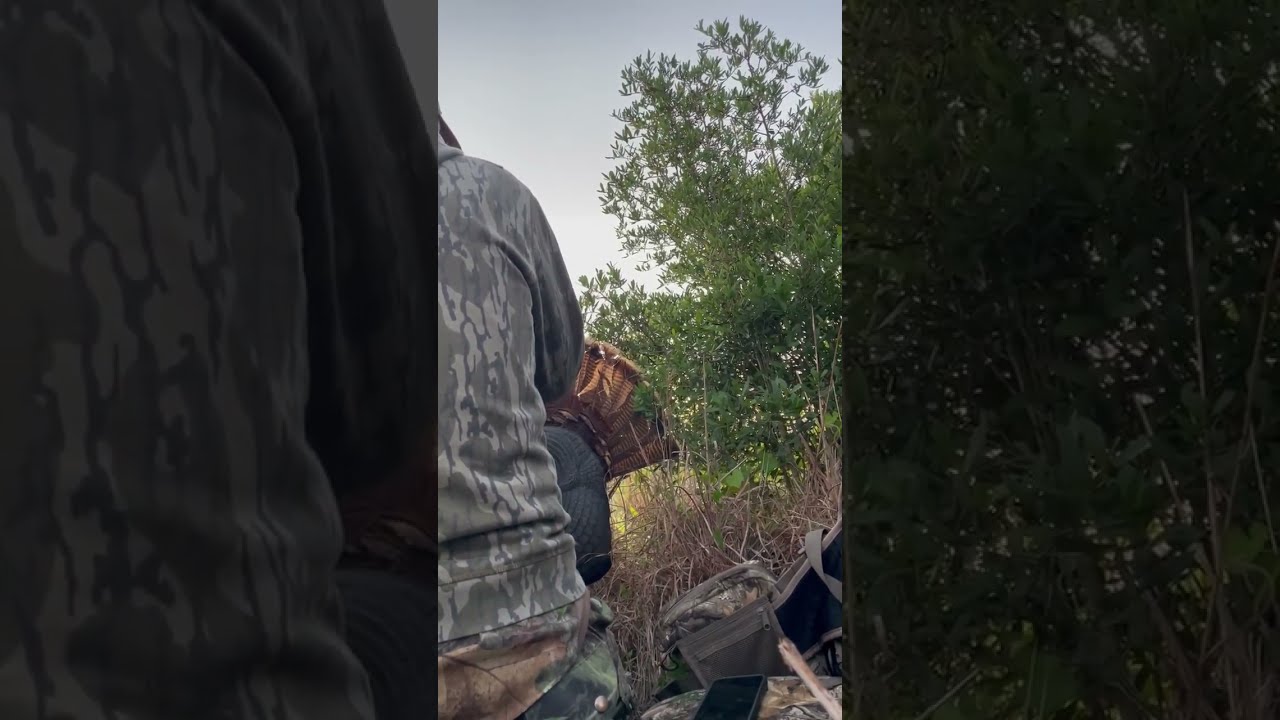The image is a six-inch wide and three-inch tall frame, divided into three sections: left, center, and right. The outer sections, which are darker, feature blown-up and darkened portions of the central image. The left section showcases a close-up of a woodland camo jacket, while the right section displays an enlarged view of trees and bushes.

In the central third, there is a detailed scene set outdoors during the daytime. The focal point is the back of an individual, who appears to be engaged in hunting. The individual is dressed in a green camouflage hoodie and pants. They are seated close to the ground, with their right shoulder and part of their back visible. The person's head is out of frame.

To the right of the individual, there is an assortment of their gear, including a camouflage backpack with a cell phone on it and another pack featuring a zipper pouch. There's also a brown woven basket nearby. The ground around them is covered in long, dead, brown grass, and above them, tall green trees and a clear blue sky are visible.

Overall, this triptych captures a serene moment outdoors, framed by complementary darkened sections that highlight the central scene without distracting from it.